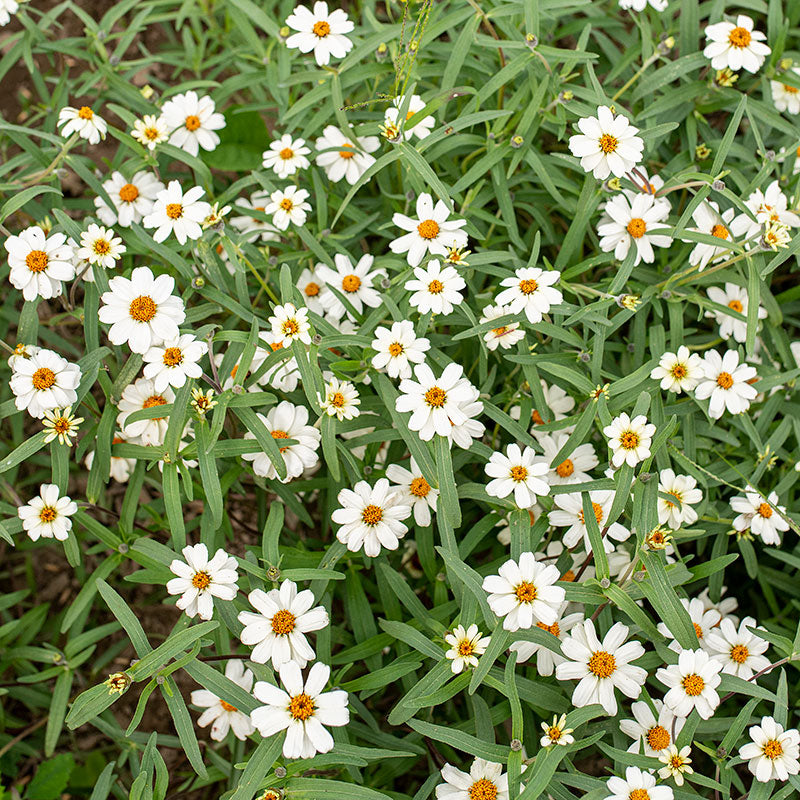This image depicts a lush field of wildflowers, specifically small daisy-like flowers with white petals and vibrant yellow centers. The flowers, each with eight to ten petals, densely populate the scene, numbering more than fifty with an abundance of green leaves interspersed throughout. The blooms stretch from the top to the bottom of the image, primarily concentrated on the left side, with the ground and some dirt visible beneath them towards the left edge. The repetitive pattern of the flowers creates a visually harmonious and natural carpet. Sunlight reflects off the petals, indicating a bright, sunny day. Notably, some bees can also be seen hovering among the blossoms, adding life to this serene natural setting.